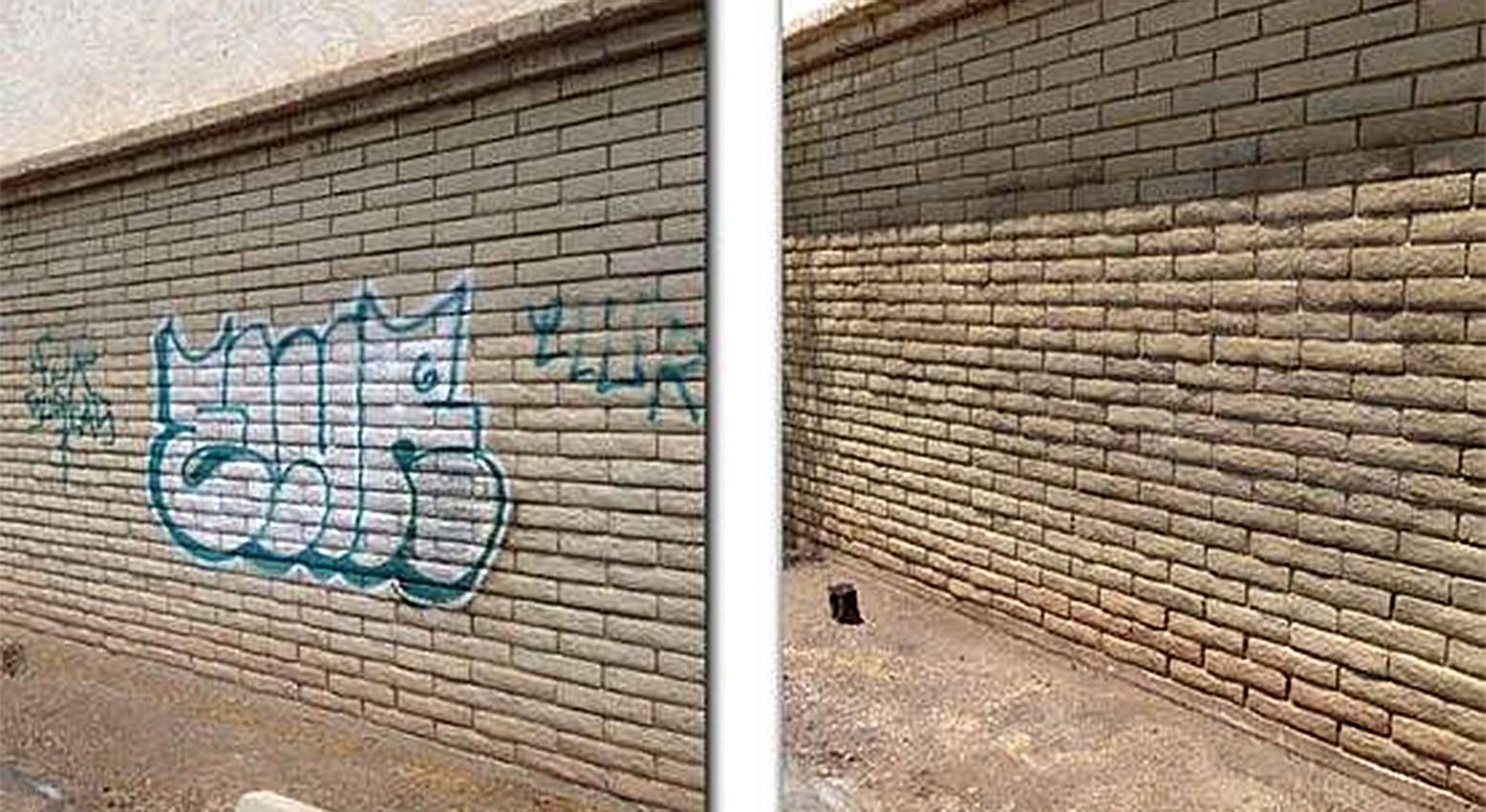The photo is an outdoor, side-by-side, before-and-after comparison of a beige sandstone-colored brick wall that has been cleaned of graffiti. The left half of the image shows the wall covered in various forms of graffiti, prominently including white bubble letters with a teal outline and tag letters that appear to spell "L-U-R" in teal. There are at least four distinct words spray-painted on the bricks, though they are not completely legible. The right half shows the same section of the wall after the graffiti has been entirely removed, revealing the natural color and texture of the brick. The wall is seen at an angle, with a dirt ground in front of it and no people or additional text in the photo. The lighting is bright and clear, indicating it was taken during the daytime. The image effectively illustrates a graffiti removal process, possibly advertising a service or project dedicated to cleaning up city spaces.